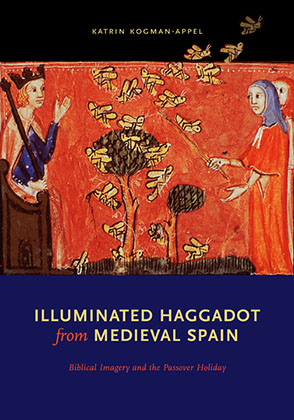This image is a detailed book cover design. At the top, there is a black bar with small yellow text reading "Katrin Kogman-Appel." The centerpiece features a medieval-style illustration on a red background. On the left side, there is a man wearing a dark blue robe and crown, holding a scepter, representing a king. To the right, there is a woman in an orange robe with a blue head shawl, holding a stick. Between them are two small trees with what appear to be yellow bees or birds flying around, and the woman seems to be swatting at the trees with her stick. The bottom third of the cover is dark blue with yellow text stating "Illuminated Haggadah from Medieval Spain," where the word "from" is highlighted in red. Below this, in smaller red text, it reads "Biblical Imagery and the Passover Holiday."